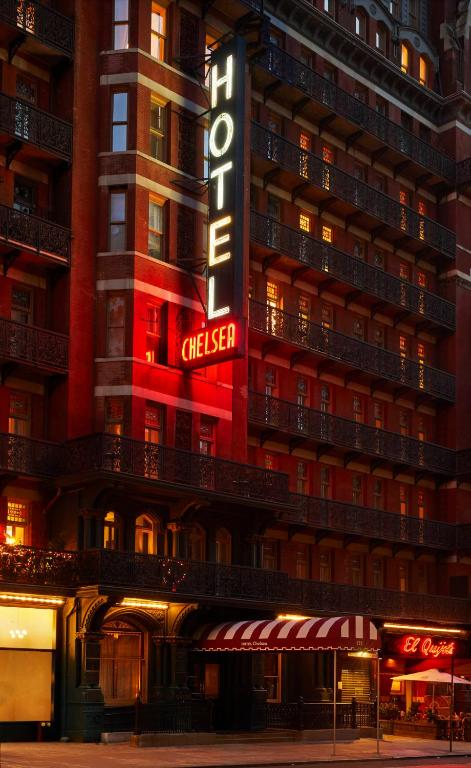The nighttime photograph captures the iconic Hotel Chelsea in a vibrant display of bright lights. The hotel, illuminated with glowing white and red signage, dominates the entire frame with its elegant structure. The building, high and distinguished, rises prominently, showing about seven stories in this close-up view. Each floor features metal balconies and numerous windows. The main entrance, adorned with a red and white canopy, sits to the left, while a blurred restaurant sign, partially legible as "LEL Q...", can be seen to the right. The scene details a purple and white awning extending from the facade under which pedestrians would pass, though none are visible. The area appears clean and well-kempt, showcasing the Hotel Chelsea as a grand and inviting establishment amid the early hours of nightfall.